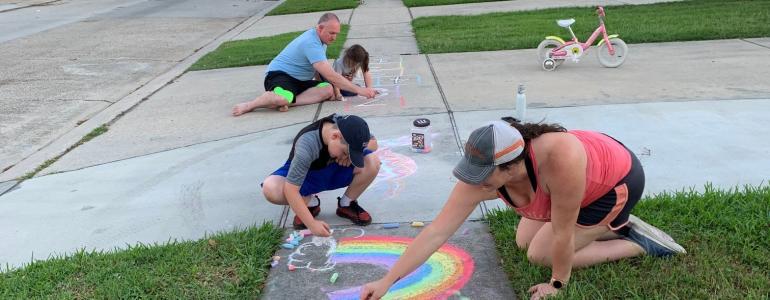In this heartwarming scene, a family of four—comprising a mother, father, daughter, and son—engages in a creative outdoor activity on an overcast day. Kneeling and sitting on the sidewalk and adjacent grassy area next to their driveway, they are deeply engrossed in drawing vibrant designs with sidewalk chalk. The mother, dressed in shorts and a t-shirt, collaborates with her young son, who sports a baseball cap, on a colorful rainbow and its adjoining clouds. Nearby, the father, barefoot and casual in lightweight attire, joins his daughter in sketching a classic hopscotch game. A pink bicycle with a white seat stands in the driveway, adding a charming touch to the backdrop. A bucket of sidewalk chalk sits prominently in the middle of the driveway, accessible to all, encapsulating the joyous essence of this artistic family bonding moment.